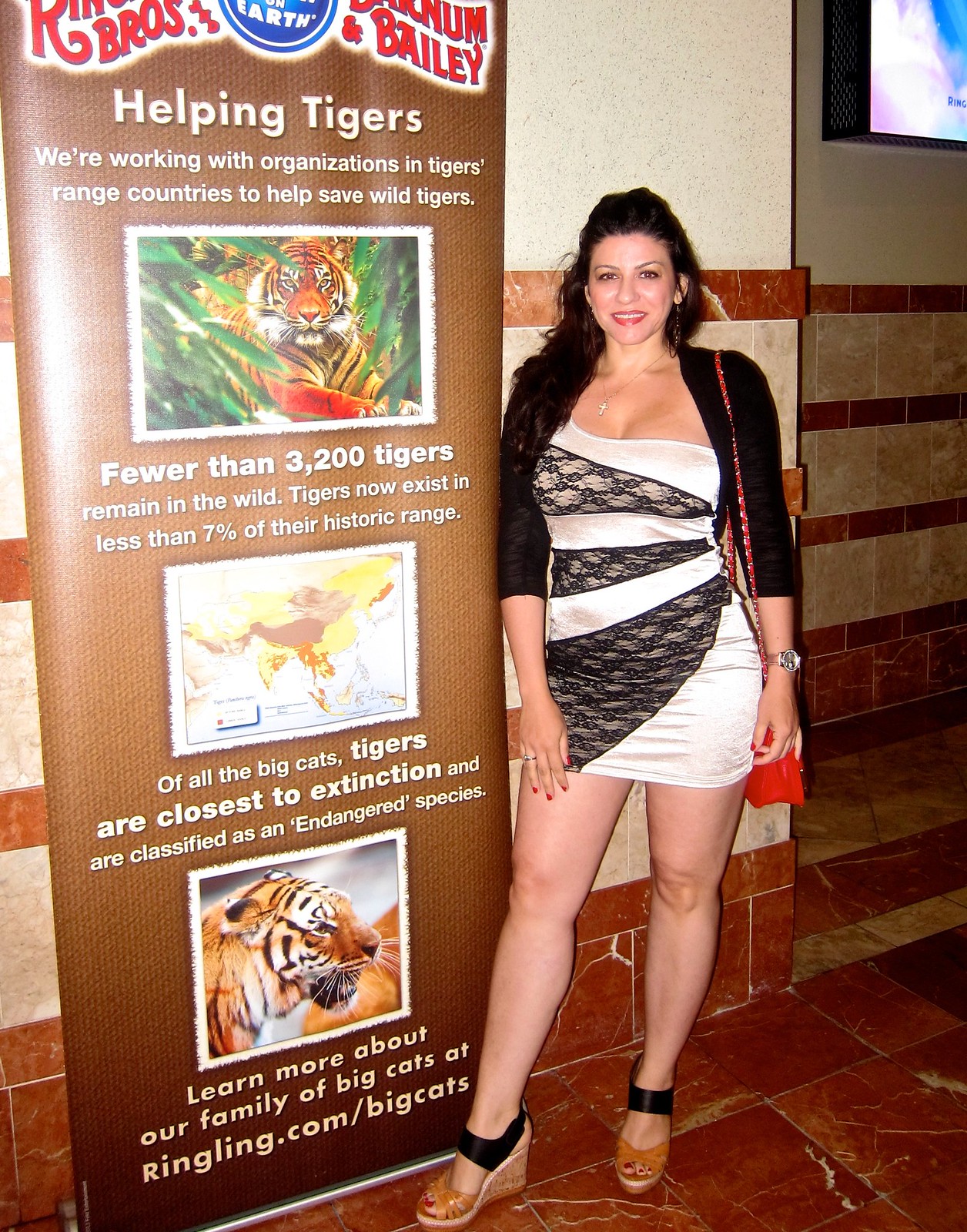The photo is a tall, rectangular image featuring a woman standing next to a narrow brown laminated sign, which is significantly taller than she is. The sign is positioned on the left side of the image, against an off-white marble wall with dark brown marble bricks running horizontally across it. The flooring consists of square dark brown marble bricks. The woman is wearing a black shawl over a white and black short dress, has dark hair, and is smiling pleasantly.

At the top of the sign, in white text, it reads "Helping Tigers." Below this heading, the sign explains that organizations in tiger-range countries are working together to help save wild tigers. The first section includes an image of a tiger surrounded by a white frame, and states, "Fewer than 3,200 tigers remain in the wild. Tigers now exist in less than 7% of their historic range." Lower down, there is a map illustrating the tigers' range and the text informs that, "Of all the big cats, tigers are closest to extinction and are classified as an endangered species." Another picture of a tiger's head is placed at the bottom of the sign. The messaging emphasizes the dire situation of wild tigers and the collaborative efforts to protect them.